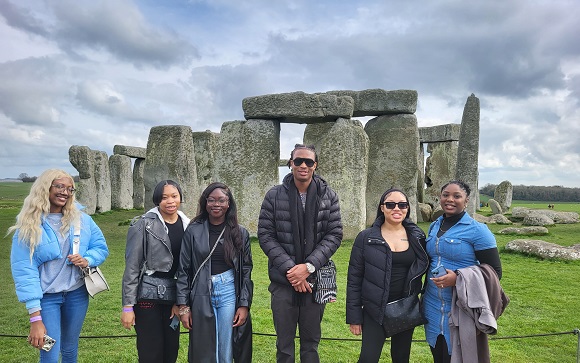A cheerful group of six tourists, all of African American descent, stand smiling for a photo in front of the iconic Stonehenge in England. The overcast sky reveals patches of blue through mostly grey clouds, casting a soft light over the scene. Stonehenge's prehistoric standing stones loom directly in the background, separated from the tourists by a rope barrier that designates the viewing area. The lawn surrounding Stonehenge is neatly trimmed. The group, dressed warmly for the chilly weather, includes a tall black man at the center, wearing an all-black puffer jacket and sunglasses, with a scarf and a watch. Flanking him are five women: to his left, one with dyed blonde hair in a blue jacket, light blue top, and dark blue jeans with a pink wristband and a white handbag; another in a black leather jacket and dress, clutching a black handbag. To his right stands a woman in a long leather trench coat, light blue jeans, and a black top; another woman in a puffer jacket, all black attire, and sunglasses; and lastly, a woman wearing a blue overdress over a black turtleneck with her jacket draped over her arms. The group radiates joy and togetherness, capturing a beautiful moment against the historic backdrop.